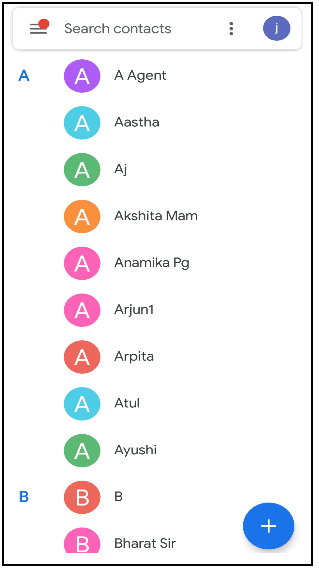In the image, which is a screenshot set against a solid white background, the heading at the top reads "Search contacts." The upper right corner of the screen features a blue circle with the lowercase letter "j" inside. On the upper left corner, there are three short horizontal lines accompanied by a red circle.

The main section of the image consists of a list of contacts, each marked with a colored circle and a corresponding letter. The contacts are displayed in the following order from top to bottom:

1. A purple circle with a white 'A' label for "A agent."
2. A blue circle with a white 'A' label for "Asta."
3. A green circle with a white 'A' label for "AJ."
4. An orange circle with a white 'A' label for "Akshita ma'am."
5. A pink circle with a white 'A' label for "Anamika PG."
6. Another pink circle with a white 'A' label for "Arjun 1."
7. A red circle with a white 'A' label for "Arpita."
8. A light blue circle with a white 'A' label for "Atul."
9. A green circle with a white 'A' label for "Ayushi."
10. A red circle with a white 'B' label for "B."
11. A pink circle with a white 'B' label for "Bharat sir."

In the lower right corner of the screen, there is a plus sign within a blue circle, likely indicating an option to add a new contact.